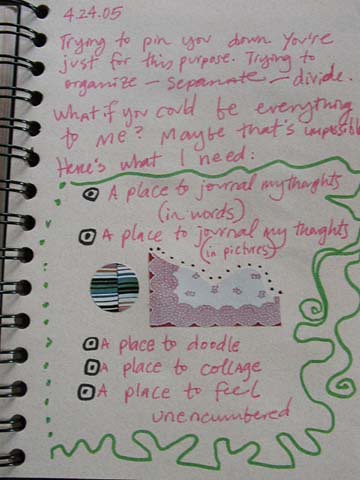The image depicts a page from a spiral-bound notebook with handwritten notes. The page, dated 04-24-05 at the top, features prominently in pink marker the phrases "trying to pin you down," and "you're just for this purpose, trying to organize, separate, divide. What if you could be everything to me? Maybe that's impossible. Here's what I need." Surrounding the text are green outlines that accentuate the writing. Below the main text, a series of bullet points, also outlined in green, lists various needs: "a place to journal my thoughts and words," "a place to journal my thoughts and pictures," "a place to doodle," "a place to collage," and "a place to feel unencumbered." The bullets are penned in black marker. The page also features some random doodles and cut-out images, indicating a creative and personal journaling process.